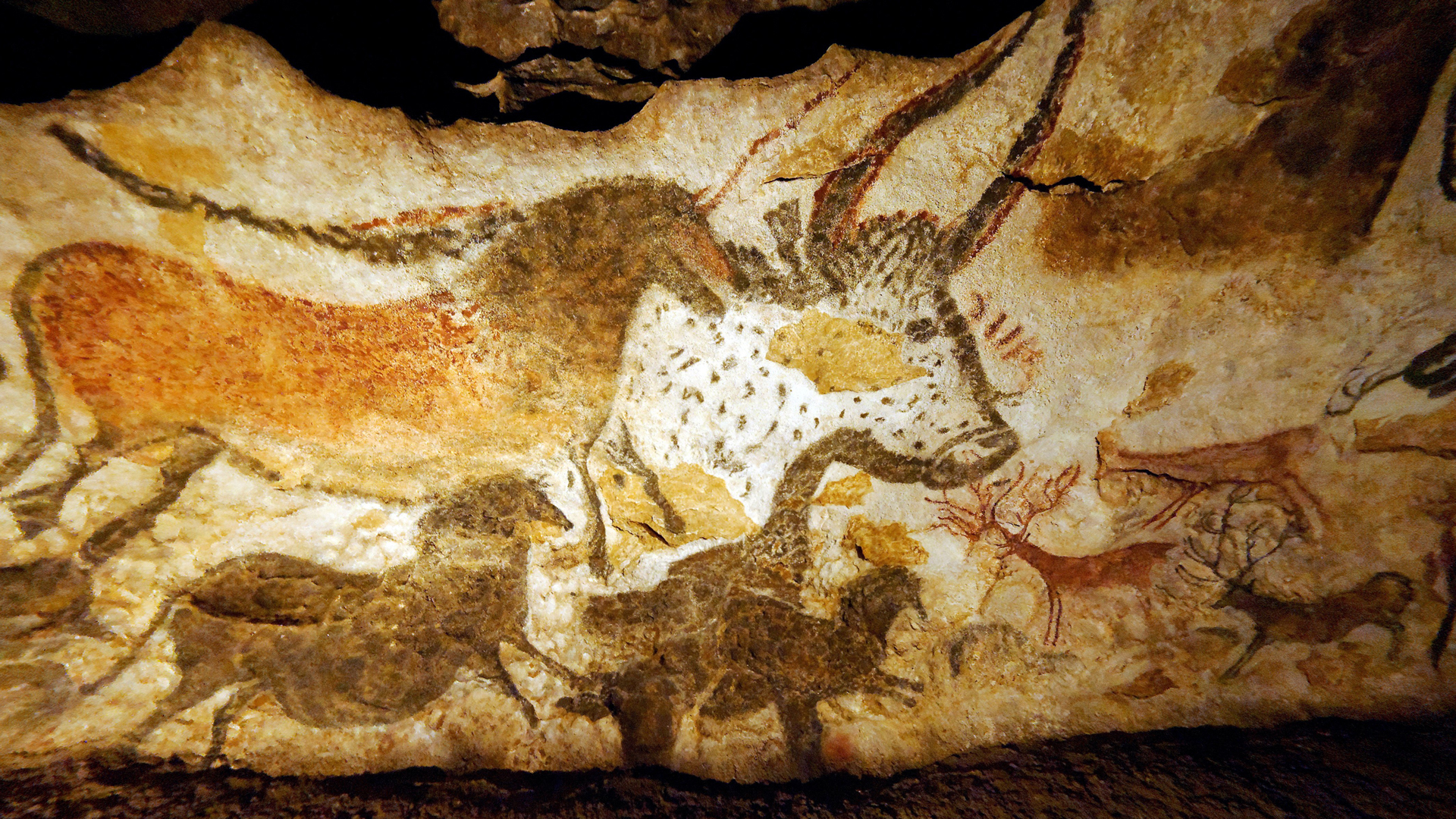This image depicts an ancient cave drawing found in European caves, showcasing a vivid representation of various wild animals. Dominating the scene is an attentive horse with an orange-brown back, a distinct mane, and a long snout. Adjacent to the horse is a striking figure of a horned animal, likely a bison or a buffalo, characterized by its white coat with brown spots and a round nose. In the backdrop, the wall carries a beige or off-white tone, providing a stark contrast to the animal figures that span the mural in shades of brown, orange, and ivory. Multiple species are featured along the bottom, all illustrated in profile, with one distinguished by a dramatic set of antlers, and others appearing low to the ground. These animals are captured in dynamic poses, suggesting movement and speed, embodying the untamed vigor of wild creatures that command respect in their natural hierarchy.